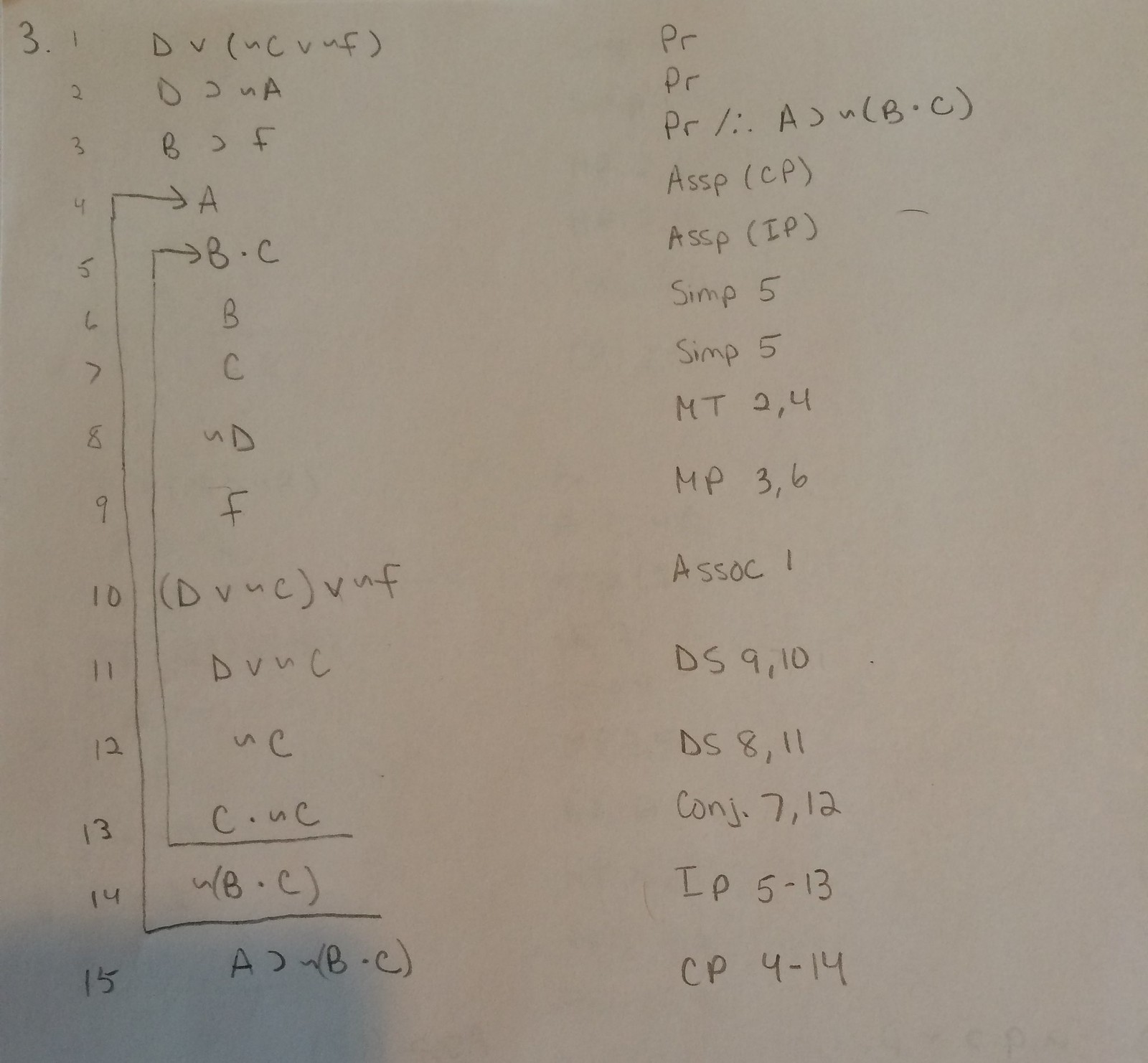This image showcases a series of 15 numbered mathematical equations, though the specific branch or type of mathematics remains unclear. Each equation is listed with its corresponding formula on the right side of the photo. The varied use of mathematical symbols, such as greater than signs, less than signs, dots, and multiplication signs, indicates a range of equation types from simple to more complex. Here is a detailed breakdown of each equation:

1. **DV**
2. **D > A**
3. **B > F**
4. **-> A**
5. **B · C**
6. **B C**
7. **C**
8. **D**
9. **F**
10. **DVC**
11. **DVC**
12. **C**
13. **C · C**
14. **B × C**
15. **A > (B × C)**

Each equation is succinctly formed, demonstrating different mathematical operations and relational expressions.